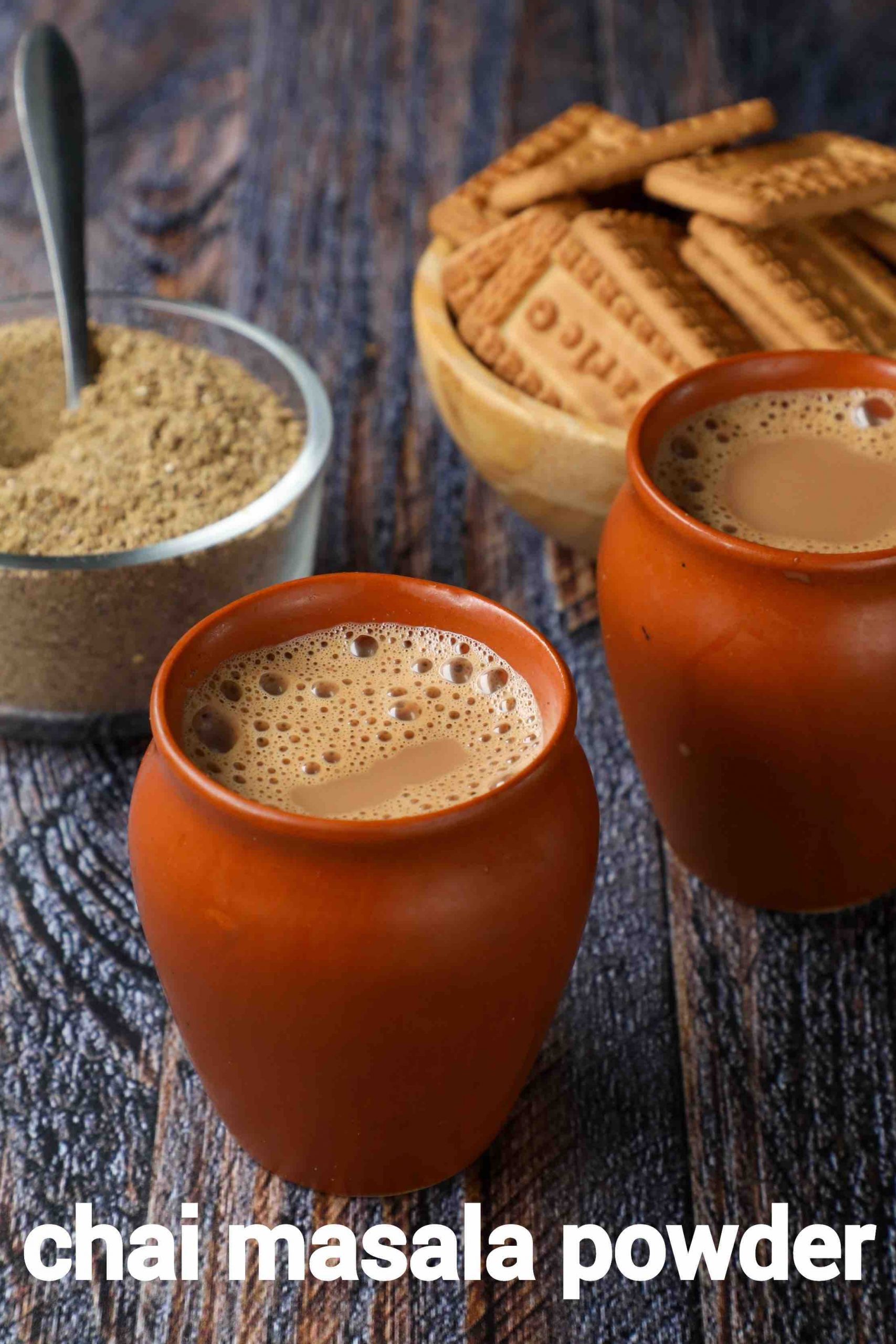The image features two terracotta-colored, vase-shaped mugs filled with a frothy, light brown liquid, possibly chai or hot chocolate, with bubbles on top. The mugs are placed on a dark, textured wooden table. Near the center, the focus is on the first mug, while the rest of the scene remains shadowed. Behind the first mug, to the top left, there's a clear, round bowl with a greenish powder inside, likely chai masala powder. To the top right, there's a tan-colored bowl filled with rectangular, heavily textured biscuits or cookies. At the bottom of the image, in large white letters, the text reads, "chai masala powder."